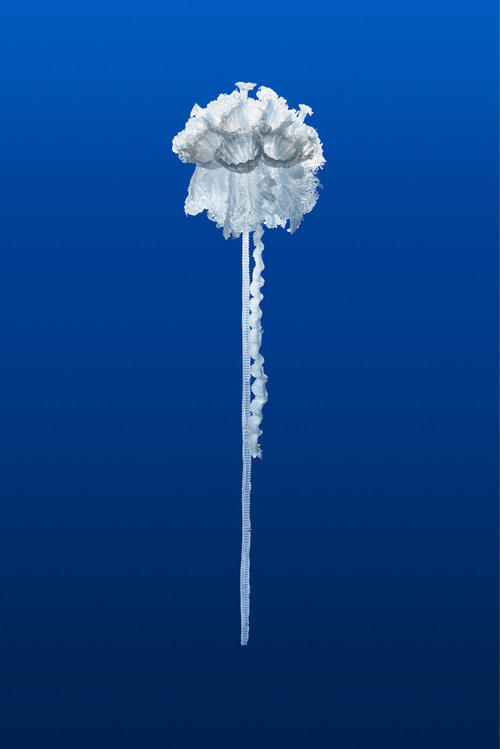Set against a deep, gradient blue backdrop that mimics the depths of the ocean, the photograph captures a large, ethereal jellyfish at its center. The jellyfish, primarily white and gray with hints of light blue, almost resembles a bloomed flower. Its top is frilly and sponge-like, enhancing its delicate and graceful appearance. The jellyfish features three bowl-shaped structures at its base, visible at the center. From its base extend two distinct tentacles: one is a long, straight line that reaches conspicuously downward, while the other is shorter and curls like a ribbon or an old telephone cord. The entire scene conveys a sense of serene suspension, as the jellyfish floats gracefully in the stillness of the deep ocean.